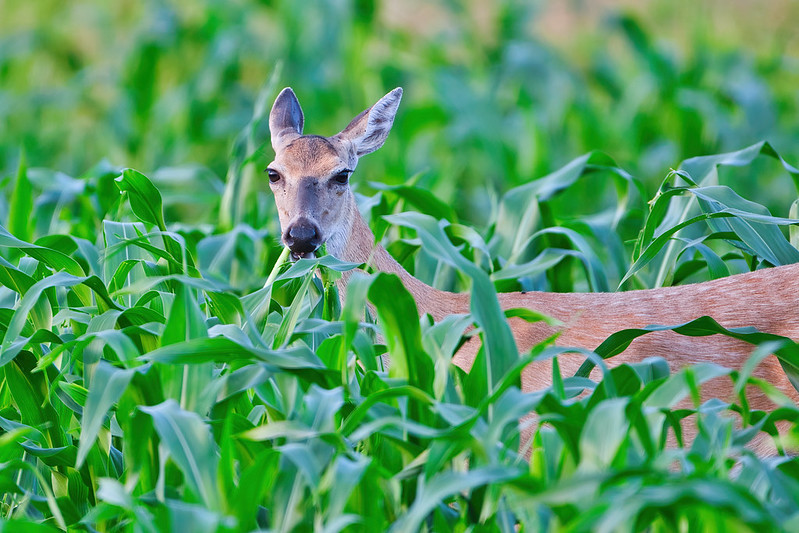The photograph depicts a vibrant landscape scene in a cornfield, captured in a landscape orientation. Dominating the image are tall, lush green corn stalks that fill the foreground and background, creating a rich, verdant setting. Amidst this sea of foliage, a deer is prominently positioned, drawing immediate attention. The deer stands among the corn stalks with its upper body and head clearly visible, while its legs are obscured by the dense greenery. It has a brown coat accented with subtle gray or whitish tones, particularly noticeable above its nose. The deer is facing the camera, its head turned frontward, showcasing its expressive black eyes framed by long, thick lashes and a pronounced black nose. Its ears are pointed upright, adding to its alert appearance. The background of the photo becomes a blur, highlighting the clarity and focus on the deer and the immediate cornfield, with daylight illuminating the scene, suggesting it is taken during the daytime.